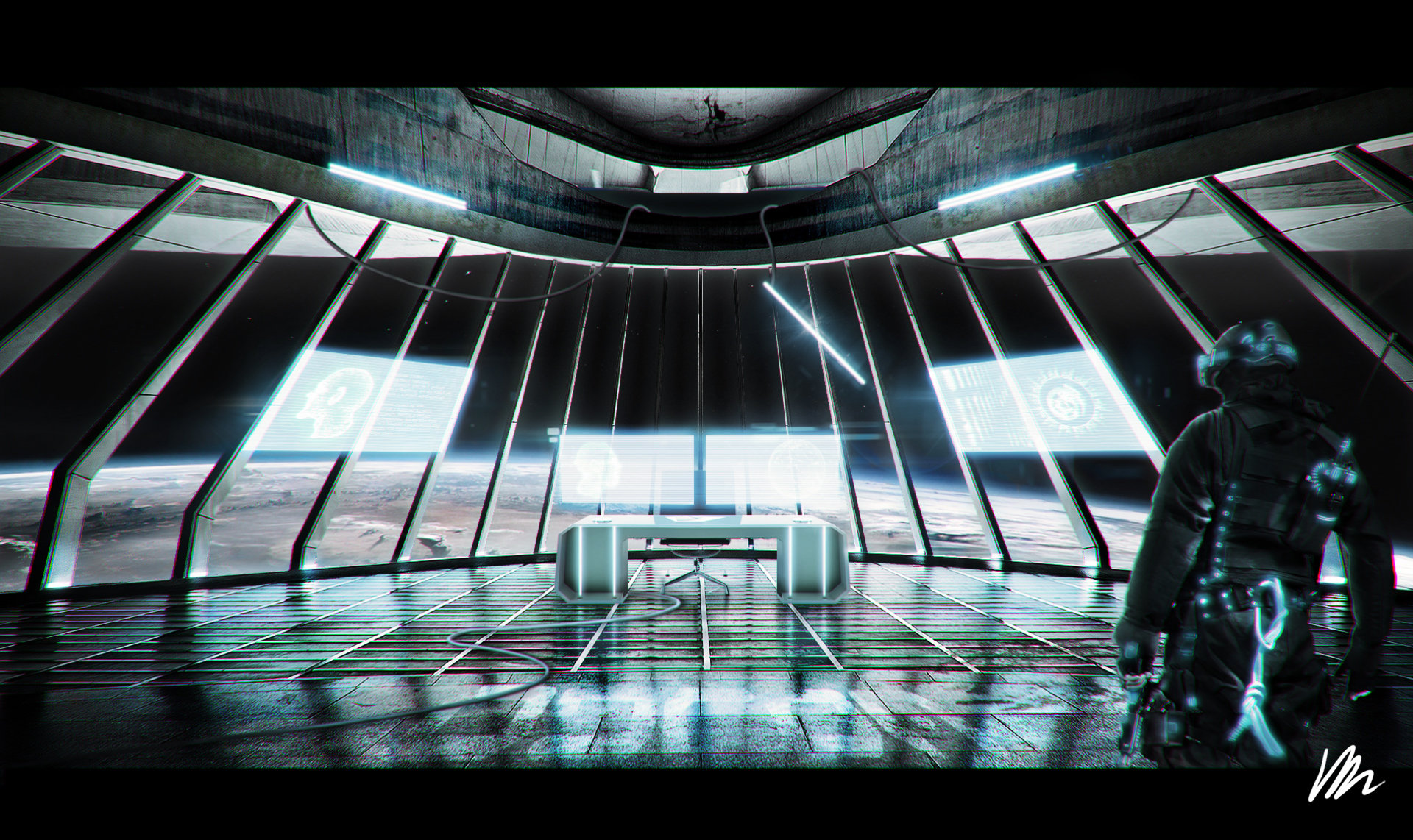In this detailed 3D rendering or painting, we find ourselves inside a futuristic command room or office within a spaceship. The room is characterized by floor-to-ceiling vertical windows framed with sturdy steel beams, offering a panoramic view of a brown, glowing planet below and the black expanse of space above. Positioned centrally, there's an empty desk accompanied by a chair, with multiple holographic monitors projected behind it and mounted on the surrounding walls with windows. A cord extends from the bottom left of the scene towards the chair, adding to the room's technological ambiance. In the bottom right corner, a slightly blurred figure in soldier-like or spacesuit gear stands thoughtfully, illuminated by glowing lights from their suit. Also notable in the corner is a white scribble, possibly indicating the artist's signature.